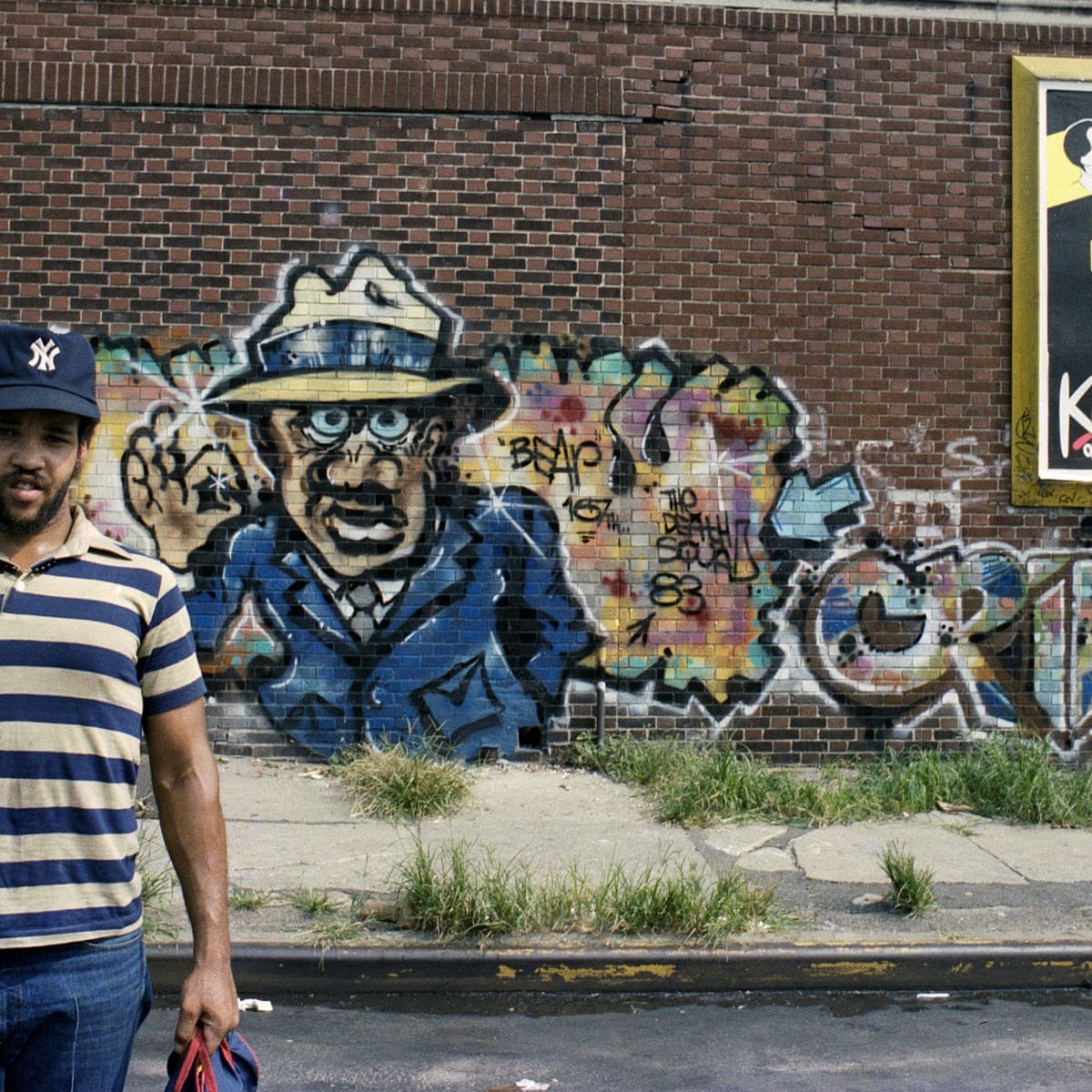This photograph captures a vivid scene of urban graffiti on the side of an old brick building. The building's dark red bricks, weathered with age, stand in sharp contrast to the overgrown grass and weeds that punctuate the neglected sidewalk in front of it. The centerpiece of the graffiti is a striking depiction of a black man in a blue suit and a light tan straw hat with a blue band. His fingers form an 'okay' gesture, radiating a sense of calm amidst the chaos. His facial features are detailed with a trimmed black mustache and mustache, and red-tinted eyes.

The artwork is set against a colorful backdrop of bright pinks, yellows, blues, and purples, adding a pop of vibrancy to the scene. Scattered throughout the mural are various names and phrases, including "To Death" and the number "83," which add layers of mystery and narrative to the artwork. 

To the right of the mural, more graffiti adorns the wall, while a figure stands out prominently on the left side of the photograph. This man, likely the artist, sports a blue and white striped collared t-shirt, a navy blue New York Yankees hat, jeans, and carries a bag that presumably holds his painting tools. His dark skin, thin black beard, and mustache mirror the features of the depicted man, adding a personal touch to this urban tableau.